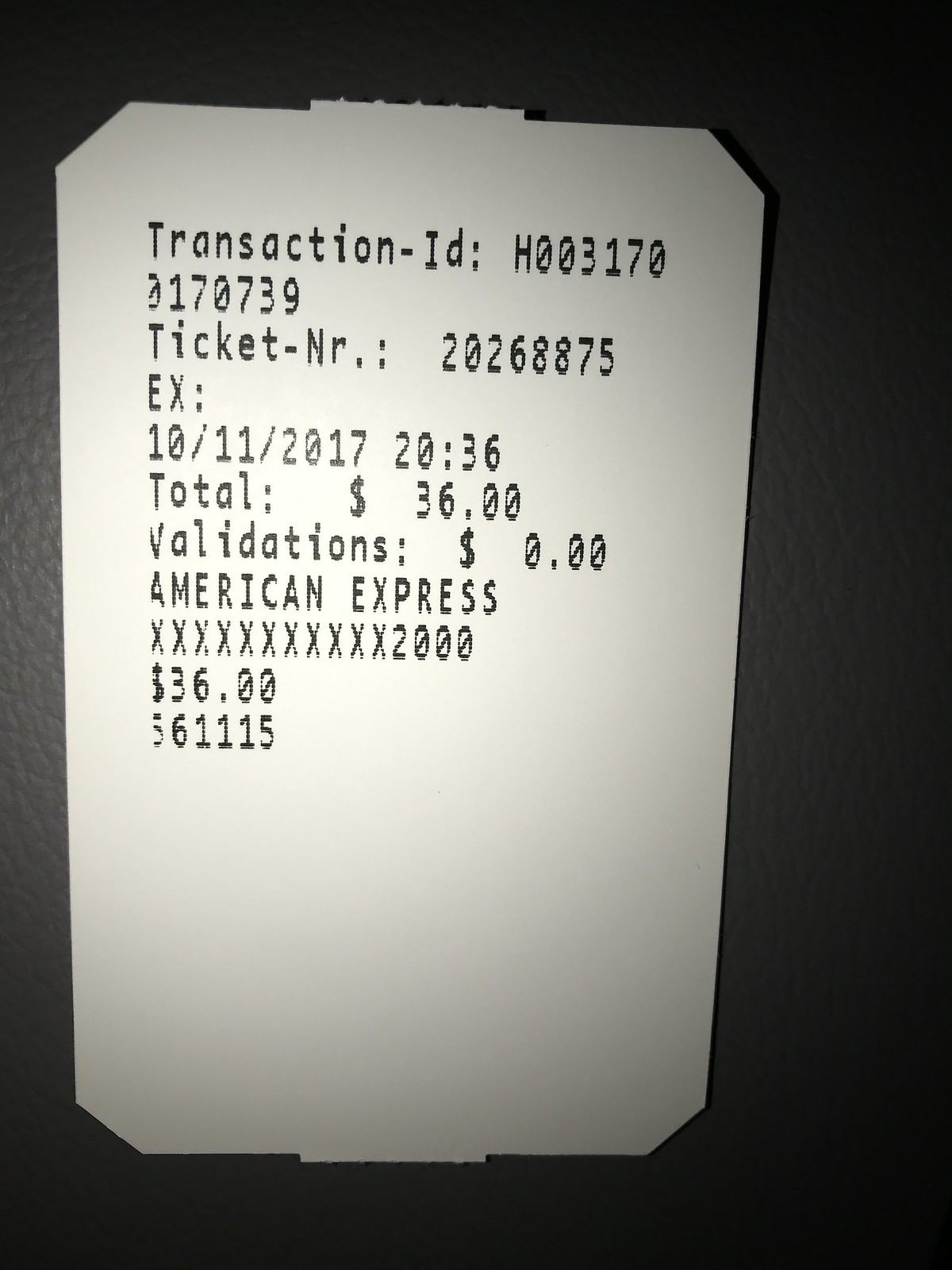A white ticket stub is displayed against a black background, revealing several important details. The ticket features a transaction ID number, a unique ticket number, and a date of October 11, 2017, with the time specified as 20:36 hours. It indicates a cost of $36, which was charged to an American Express card ending in 2000. The ticket is very plain and does not specify the event or purpose it was issued for. On either end of the stub, there are small perforations near the center, indicating it was detached from adjacent tickets.